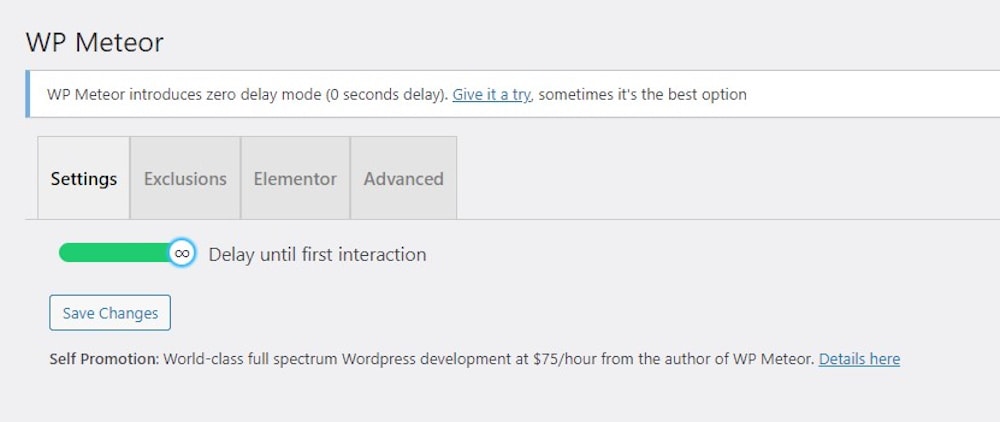The screenshot portrays a segment of a WordPress admin page with a light gray background, indicating it might be for utility or settings configuration on a website. The top left corner features the text "WP METEOR" in black capital letters, suggesting it is related to the WP Meteor plugin. Beneath this title, there's a white rectangular box with a light gray font reading, "WP Meteor introduces zero delay mode (zero second delay), give it a try." The phrase "give it a try" is underlined and blue, signaling it as a clickable hyperlink. 

Below this are four square icons labeled: Settings, Exclusions, Elementor, and Advanced, corresponding to different configurable options within the plugin. A short green line with a white circle at its right end lies below the squares, alongside the text "Delay until first interaction."

Further down is a white button with light bluish-gray text saying "Save Changes." At the very bottom, another section against the light gray background promotes the author's services: "Self-promotion: world-class full-spectrum WordPress development at $75 an hour from the author of WP Meteor." The phrase "details here" is underlined and in blue, indicating another hyperlink.